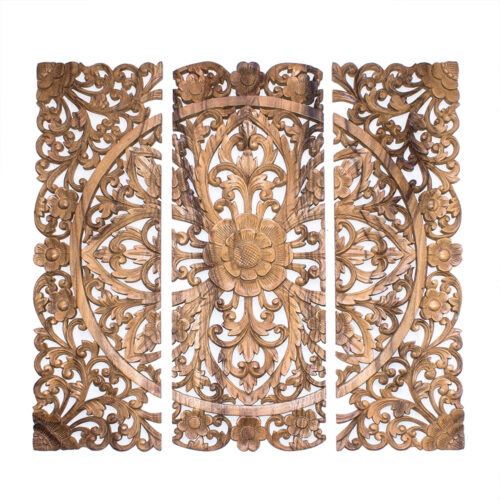The image showcases an ornately carved wooden decorative piece, likely a room divider or screen, consisting of three wooden panels. The wood is a light to medium brown with a slightly glossy finish. The panels are intricately designed with a lace-like pattern that maintains a consistent decoration across each segment. At the center of the combined panels is a circular motif that spans all three sections, featuring a central flower with large petals, giving it a mandala-like appearance. The floral design is detailed and symmetrical, with botanical embellishments such as vines, smaller flowers, and leaves carved into the wood. The carving is pierced all the way through, creating an airy, see-through effect. The photograph has a clean, simple background, either transparent or white, which highlights the detailed craftsmanship of the wooden piece.